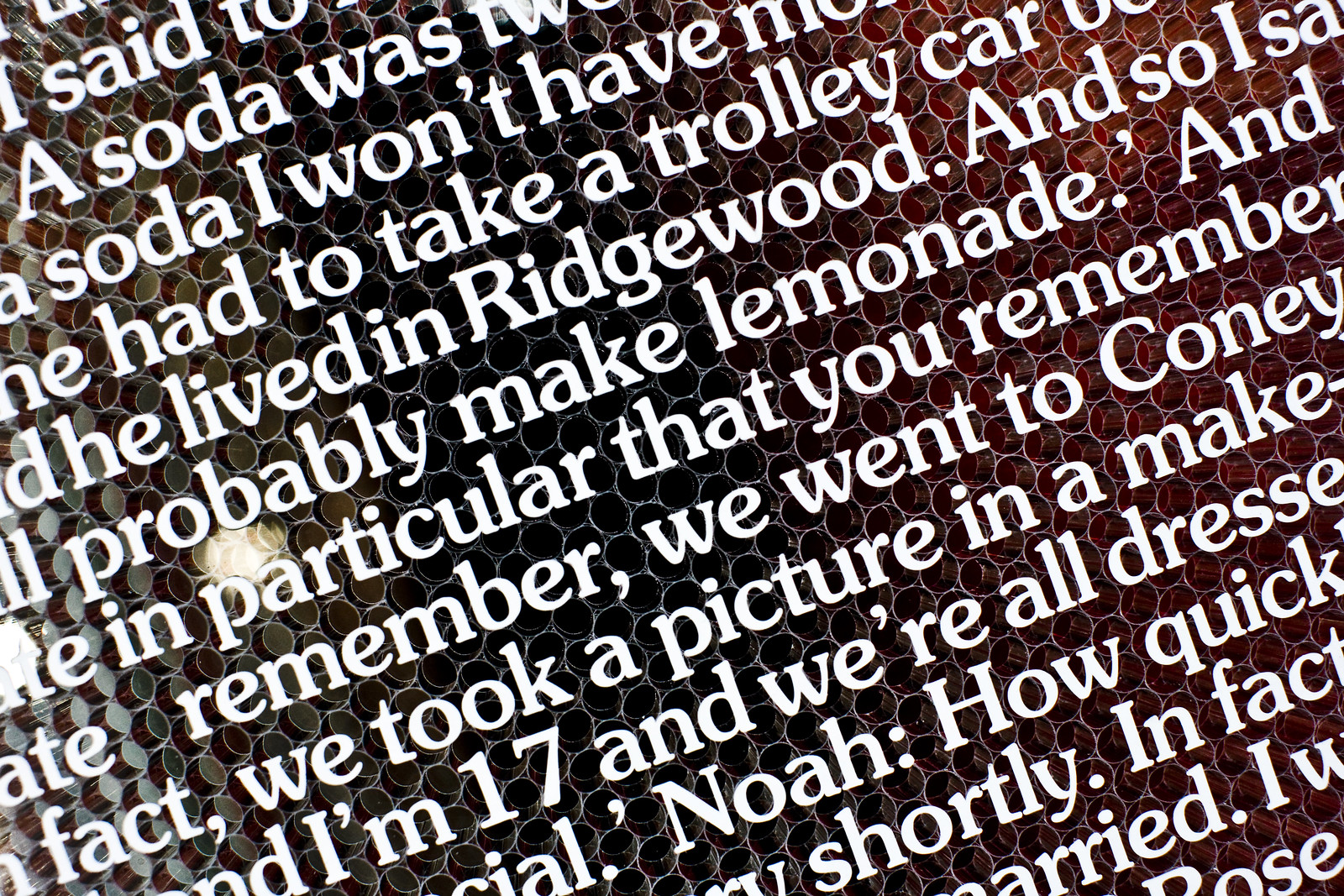An image with an all-black background featuring scattered circles in varying colors—red on the right, white on the left, and splashes of brown, pink, or blue. Amidst the colorful circles, fragmented, white, diagonal text is strewn across the image. Though disjointed, snippets of text read: “a soda was to a Soda,” “I won’t have mo...,” “had to take a trolley car,” “he lived in Ridgewood,” “probably make lemonade,” and “remember we took a picture.” Other text includes, “I’m 17 and we’re all dressed special,” and mentions of Noah, marriage, and a nostalgic recollection, reflecting a chaotic yet intimate snapshot of fragmented memories.